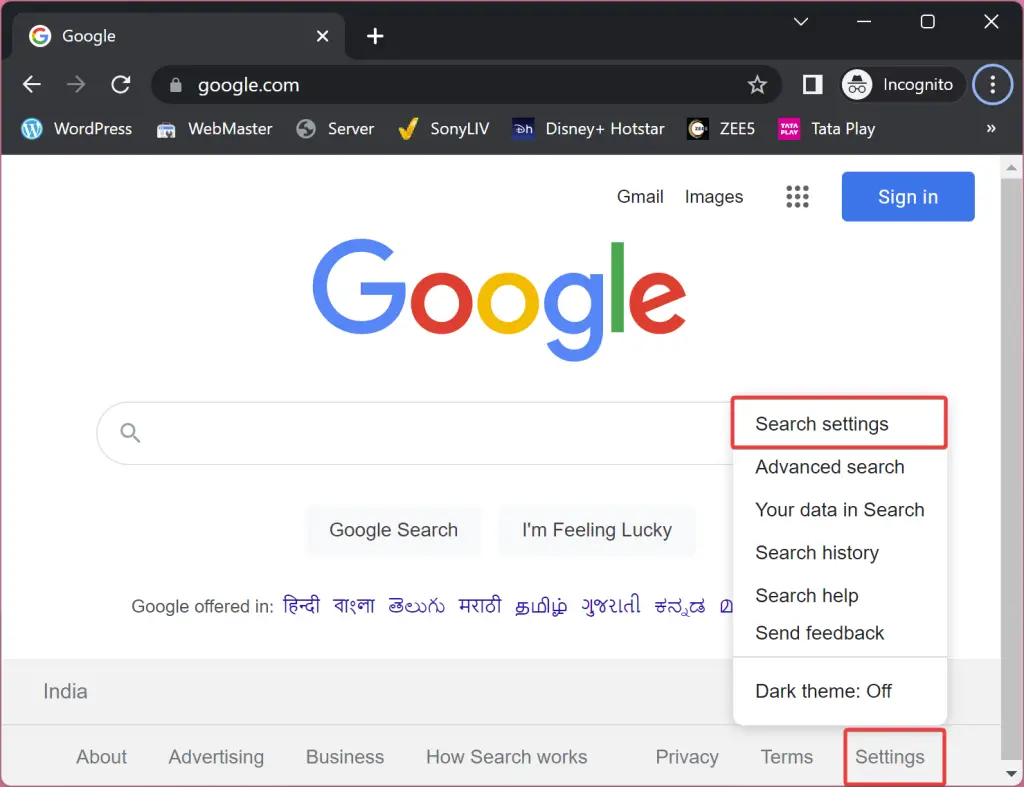The screenshot captures a typical Google homepage within a web browser operating in incognito mode. The central focus is the unmistakable colorful Google logo situated above the classic search bar, which remains empty. Below the search bar, the standard "Google Search" and "I'm Feeling Lucky" buttons are prominently displayed. 

To the right side of the screen, a settings panel is highlighted in red, making options such as "Advanced search," "Your data in Search," "Search history," "Search help," "Send feedback," and "Dark theme: off" visible. Below this panel, another "Settings" label is also highlighted in red.

On the left side of the highlighted settings, there are links labeled "Terms," "Privacy," "How Search Works," "Business," "Advertising," followed by "About." Above the "About" section, the page indicates the user's region with "India" and a line stating "Google offered in" followed by text in a script resembling the Indian alphabet.

At the top of the page, the upper navigation bar features options for "Gmail" and "Images," along with a grid icon that provides access to various Google apps. There is also a prominent blue "Sign in" button to the right.

The browser interface reveals several bookmarks with recognizable icons and labels for WordPress, Webmaster, Server, Sony LIV, Disney+ Hotstar, Zs, and Tata Play. Above the bookmarks bar, an incognito mode icon is visible, indicating the user's private browsing session.